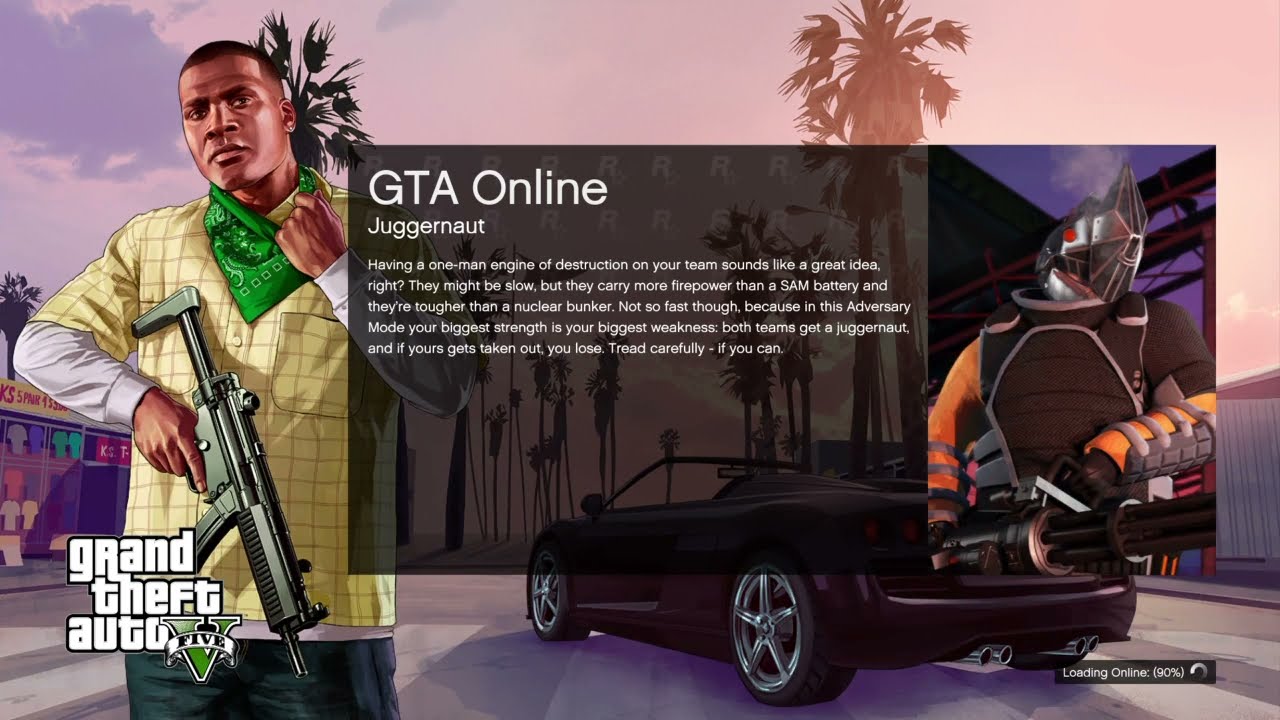This is a detailed screenshot from the loading screen of Grand Theft Auto 5's online mode. Dominating the center of the image is a rectangular text box with essential game information in white font. It reads: "GTA Online Juggernaut: Having a one-man engine of destruction on your team sounds like a great idea, right? They might be slow, but they carry more firepower than an SAM battery, and they're tougher than a nuclear bunker. Not so fast though, because in the adversary mode, your biggest strength is your biggest weakness. Both teams get a juggernaut, and if yours gets taken out, you lose. Tread carefully if you can."

On the left-hand side of the image, a dark-skinned man is depicted. He has short black hair and is wearing a yellow checkered polo over a white long-sleeve shirt, blue jeans, and a lime green bandana. He holds a black automatic gun pointed downwards. Behind him on the far left is a vibrant t-shirt kiosk displaying shirts in colors like orange, yellow, purple, and turquoise.

To the right of the text box stands the juggernaut. Clad in contrasting orange and black armor, the juggernaut has a silver, knight-like helmet and wields a massive, black Gatling gun. The car, colored magenta, is situated towards the bottom center of the image, set against a backdrop of scattered palm trees and a sky with purplish-blue hues. The bottom left corner of the image prominently features the text "Grand Theft Auto 5," while the bottom right corner shows "loading online at 90%."